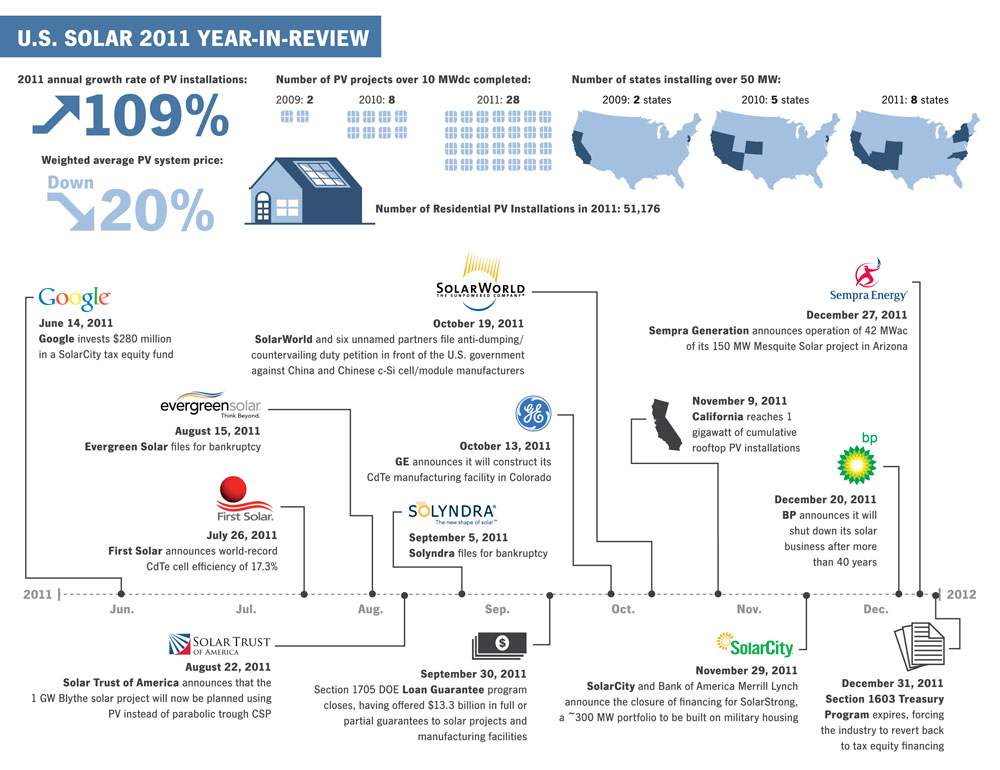**Diagram Description: U.S. Solar 2011 Year in Review**

The diagram offers a detailed review of the U.S. solar industry's performance and key events in 2011. This visual presentation is predominantly white, with black and blue text, featuring two distinct shades of blue for various illustrations. At the top, a blue banner with white letters reads, "U.S. Solar, 2011 Year in Review." 

Below this, in black letters, it states, "2011 Annual Growth Rate of PV Installations," accompanied by a blue arrow pointing to the right with "109%" in blue inside the arrow. To the right, the text reads, "Number of PV projects over 10 MW DC completed," with numbers detailing progress over the years - "2009: 2", "2010: 6", and "2011: 28" - displayed alongside small blue dots.

Three maps of the United States illustrate the expansion of solar installations. For 2009, two states (centered around California) are highlighted. The map for 2010 shows five states, extending slightly south and east. By 2011, eight states are marked, including California, the upper Northeast, and Central East regions, indicating an increasing number of states installing over 50 MW of solar power.

Key events are highlighted below the maps, each marked with specific dates:

- **Google (June 14, 2011)**: Google invests $280 million in a SolarCity tax equity fund.
- **Evergreen Solar (August 15, 2011)**: Evergreen Solar files for bankruptcy.
- **First Solar (July 26, 2011)**: Announces a world record for cell efficiency at 17.3%.
- **SolarWorld (Various dates)**: Notable strategic updates with significant dates.
- **GE (October 13, 2011)**: Key developments in solar technology.
- **Solyndra (September 5, 2011)**: Files for bankruptcy.
- **Sumtra Energy (December 27, 2011)**: Updates in solar projects.
- **BP Gasoline (December 20, 2011)**: Engagements in solar energy projects.
- **California (November 10, 2011)**: Reaches one gigawatt of cumulative rooftop PV installations.

Additional details at the bottom include:

- **SolarTrust (August 22, 2011)**: Strategic movements.
- **Monetary developments (September 30, 2011)**.
- **SolarCity (November 29, 2011)**: Key installations and investments.
- **Section 1603, Treasury Program (December 31, 2011)**: Financial incentives and impacts.

A notable visual at the top-right corner showcases a house icon with an arrow indicating a decrease of 20%, detailing the number of residential PV installations in 2011, marked at 51,176.

Overall, this diagram presents a comprehensive and chronological overview of the pivotal moments, growth trends, and key financial movements within the U.S. solar industry throughout 2011.